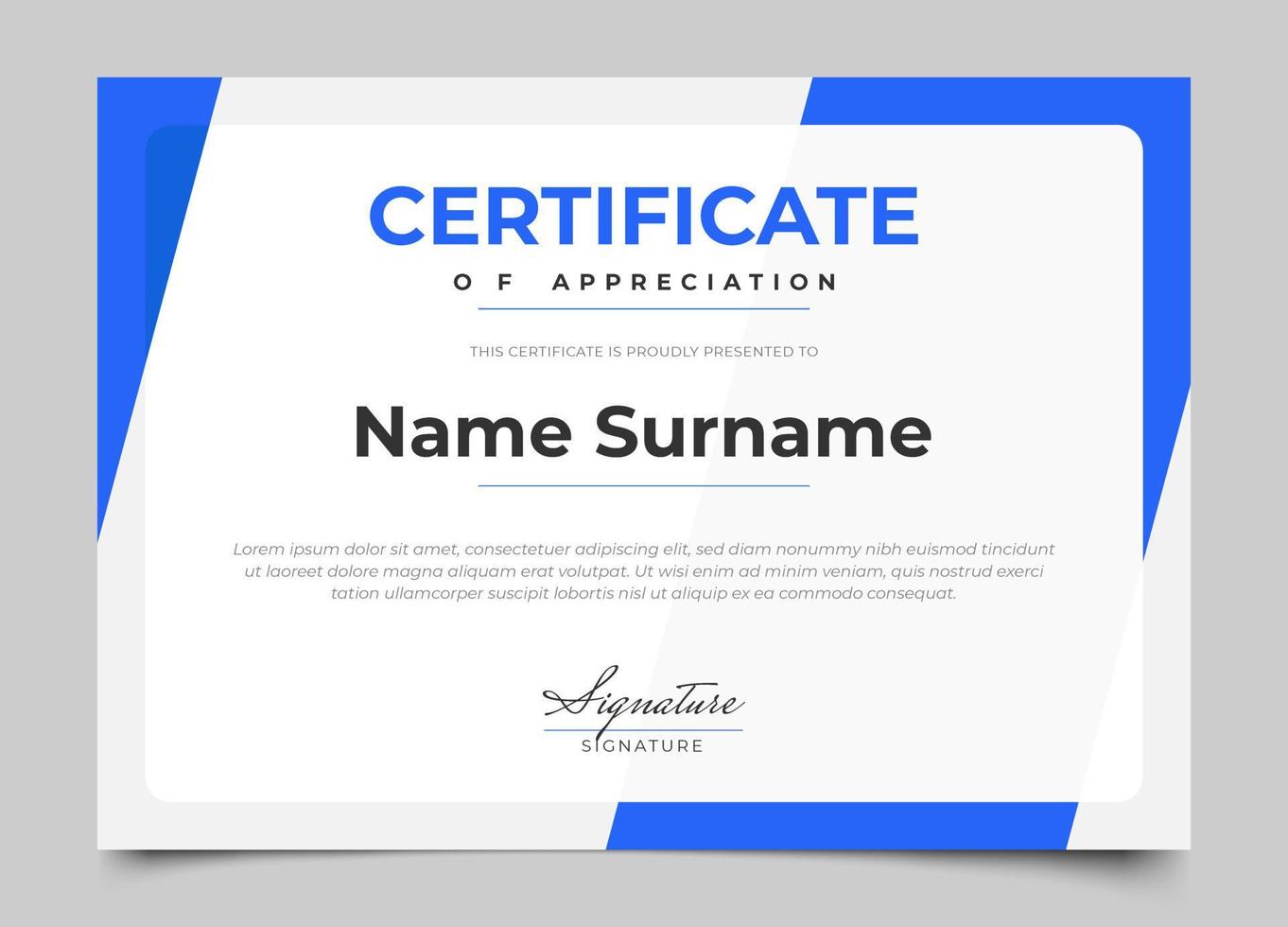The image is a horizontally oriented digital representation or mock sample of a certificate of appreciation set against a gray background. The certificate itself features a white background adorned with blue edges and decorative elements. Prominently, in the upper middle section, the text "Certificate of Appreciation" is displayed in blue and black font. Below this, there is a blue bar, followed by the phrase "This certificate is proudly presented to" in a lighter gray font. A placeholder text "Name, Surname" in black font indicates where the recipient's name should be filled in. Further down, there is an area filled with what appears to be placeholder text in Latin, commonly known as "Lorem Ipsum," used to demonstrate the layout of text. At the bottom of the certificate, the word "Signature" is shown in a signature font, with a space labeled "Signature" in plain text below it, designated for the actual signing. This template serves as a formal indication of the final design for those interested in creating a personalized certificate of appreciation.